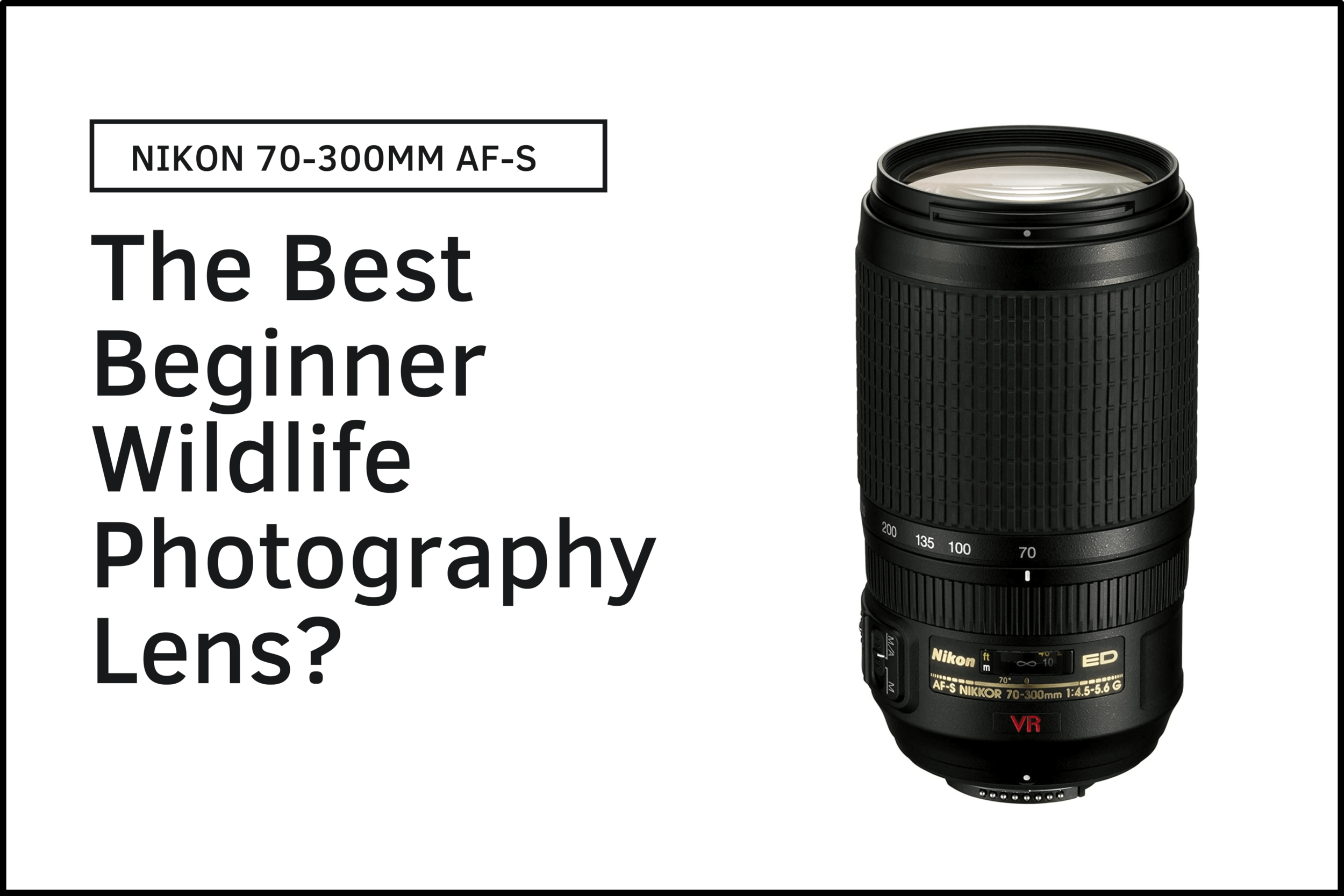The image features a Nikon 70-300mm AF-S lens standing upright with the lens facing the top of the image. The lens is predominantly black with a gold "Nikon" logo near the bottom of its cylindrical shape, along with other details like "AF-S" and "VR" in red further down. The background of the image is white, bordered by a thin black line, creating a clean and focused presentation. On the left side of the image, black text on a white background reads “Nikon 70-300mm AF-S” inside a rectangle lined box, followed by the larger question in black text, “The best beginner wildlife photography lens?” The overall layout is rectangular, slightly wider than it is tall, with text on the left side and the image of the lens on the right, highlighting various features and numbers pertinent to the lens’s specifications, such as 201, 135, 170, and 70-300mm.